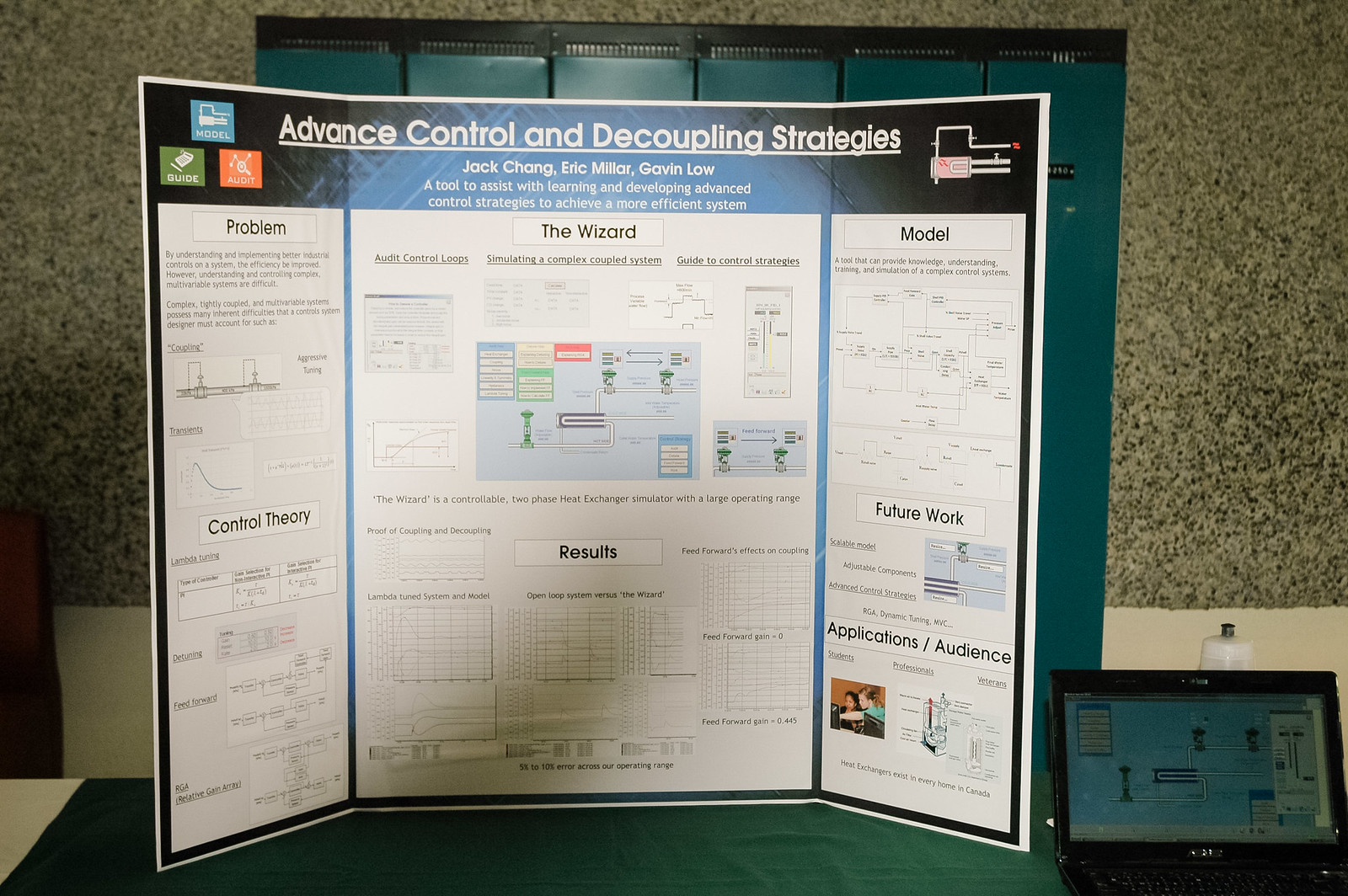The photograph showcases a detailed presentation on a large tri-fold poster board set against a speckled gray wall with a darker green section in the center. The poster board, which has a white border, bears the headline "Advanced Control and Decoupling Strategies" in bold white font, underlined at the top. Directly below the title are the names "Jack Chang, Eric Miller, and Gavin Lowe."

The poster is organized into three distinct panels:

1. **Left Panel**: 
   - Title: "Problem Control Theory"
   - Features three colored squares in the upper left corner: a blue square labeled "Model," a green square labeled "Guide," and an orange square labeled "Audit."

2. **Center Panel**: 
   - Title: "The Wizard and Results"
   - Contains subsections such as "Audit Control Loops," "Simulating a Complex Coupled System," and "Guide to Control Strategies," each with illustrative diagrams and images below.

3. **Right Panel**: 
   - Titles: "Model," "Future Work and Applications," and "Audience"
   - Each section includes descriptions and small diagrams, which are hard to discern clearly.

Additional elements include a tabletop draped with a green cover, a black iPad on the lower right corner displaying a blue diagram, and a schematic drawing near the top of the right panel. The overall display appears to be an educational tool designed to assist with learning and developing advanced control strategies for more efficient systems.